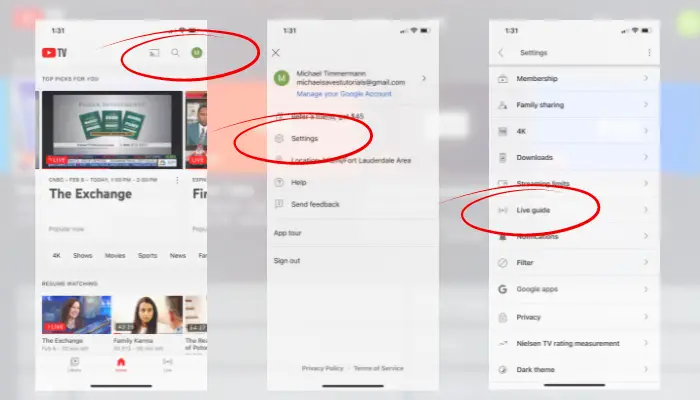Here is your cleaned-up and detailed caption:

---

This composite image consists of three smartphone screenshots arranged vertically, each highlighted to guide the viewer through a specific sequence. 

1. **First Screenshot (Top):**
   - **Header:** The upper left corner displays the current time, while the upper right corner indicates the Wi-Fi signal strength and battery percentage.
   - **Main Body:** A YouTube TV icon is prominently featured at the top. A red circular highlight, resembling a highlighter mark, draws attention to a particular section of the screen. Below this, there is a photograph labeled "The Exchange." Further down, several filtering options are visible, and at the very bottom, three video thumbnails are displayed.

2. **Second Screenshot (Middle):**
   - **Main Body:** Similar to the first screenshot, this one also includes a red highlighter-style circle. This time, the circle emphasizes the settings option, suggesting its importance in the sequence.

3. **Third Screenshot (Bottom):**
   - **Main Body:** Continuing the highlighted guidance, the red highlighter marks the "Live Guide" option. This indicates the final step in the process, directing the viewer on how to access the live guide feature.

Overall, the series of screenshots instructs the user through a step-by-step process: 
1. Identifying a specific part of the YouTube TV interface.
2. Navigating to the settings.
3. Accessing the live guide feature.